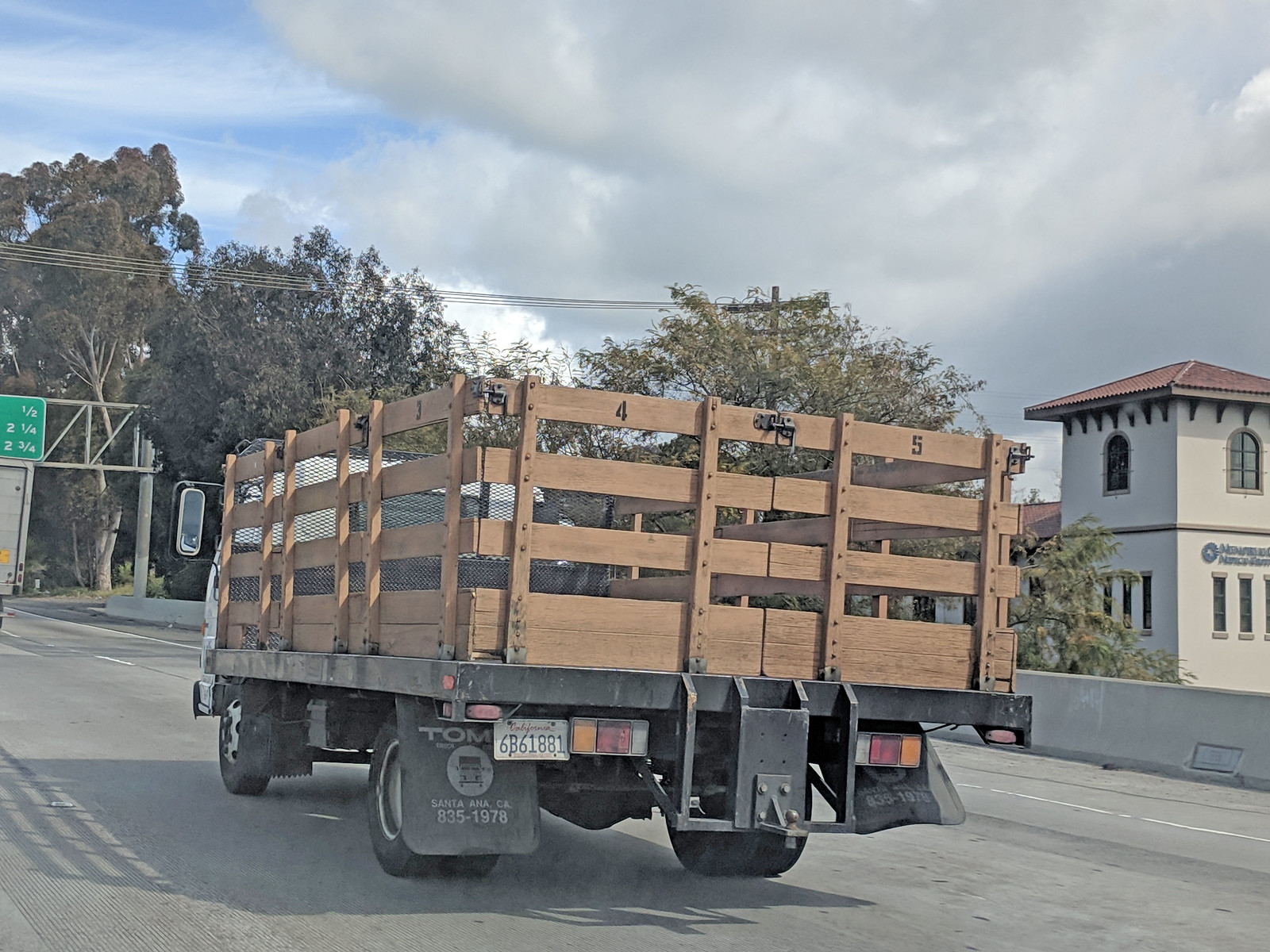This is an angled photograph of the back of a large commercial-sized box truck driving down a multi-lane road or highway. The truck has a flatbed with a wooden rail frame that looks like a fencing enclosure, enclosing the bed. The wooden frame is sectioned and numbered, with visible numbers including 3, 4, and 5. Some descriptions mention the numbers 6, 7, and 8 on the other side. The frame is lined with some form of netting or metal fencing.

The truck has a California license plate with the number 6B61881 and mud flaps over the rear tires; the right mud flap is flapping in the wind and bears the text "Tom, Santa Ana, California 835-1978." There are two tail lights with three horizontal lights each: orange, red, and white, although the right tail light is partially obscured by a metal hitch with a towing ball on the back.

Through the wooden slats of the frame, you can see that the cab of the truck is white. The vehicles and structures in the background suggest a scenic route, possibly in California, characterized by Mediterranean-style architecture. A two-story building with a terracotta-tiled roof and arched windows is visible on the right side, alongside trees and a concrete barrier or divider. The weather appears varied, with a blue sky partly covered by dark, fluffy clouds. Telephone poles and wires cross above the road, adding to the contextual atmosphere of a typical American roadway. There's also a green highway sign with mileage markers that reads "1/2," "2 1/4," and "2 3/4" indicating distances to upcoming exits or locations. This detailed setup portrays a dynamic truck scene on a U.S. highway, traveling through a visually descriptive and characteristic landscape.